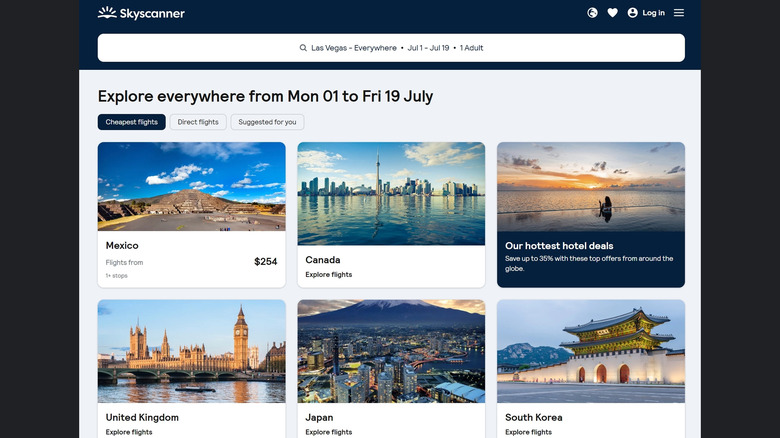The image showcases a travel website interface, likely captured from a laptop screen. The primary backdrop is black, punctuated by sections with white backgrounds that display various elements. 

In the upper left-hand corner, the first visible element is a "SkyScanner" logo featuring a small sun illustration. The upper right-hand corner contains icons, along with a "Log in" option. Just below this is a search bar enclosed within a rounded-corner rectangle, displaying in very small font: "Las Vegas everywhere July 1st to July 19th one adult."

The subsequent section is dominated by a large white rectangle. The top row within this area states: "Explore everywhere from Monday 01 to Friday 19 July." Below this are three buttons labeled "Cheapest flights" (highlighted in blue), "Direct flights," and "Suggested for you."

Following this, there are two rows, each containing three boxes with rounded corners and images on top. In the first row, the boxes are titled "Mexico flights from 254," "Canada explore flights," and "Our hottest hotel deals save up to 35% with these top offers from around the globe" (the last one highlighted in blue). The second row features "United Kingdom," "Japan," and "South Korea," each with corresponding images.